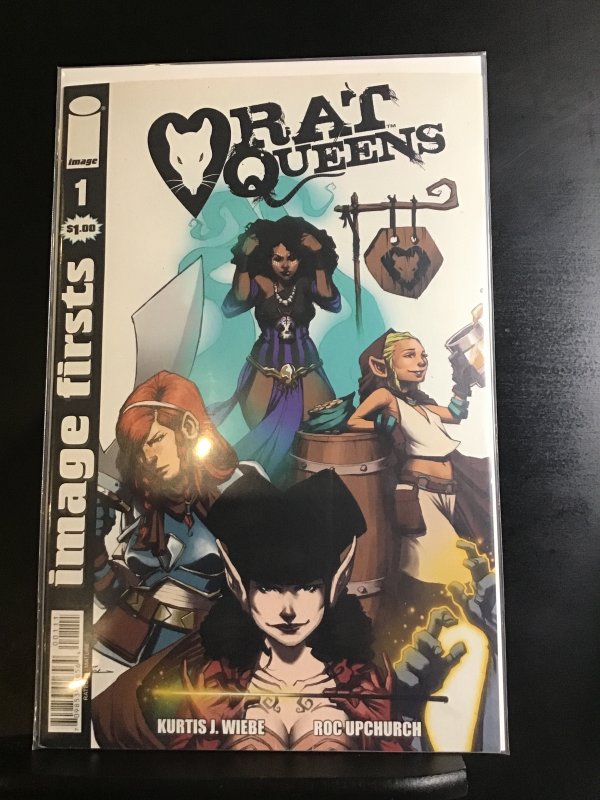The image is a detailed magazine cover with an anime-comic style, entitled "Rat Queens," featuring a rat's face icon in white. A diverse group of female characters is prominently displayed. At the top, there is a Black woman with big black hair, wearing a purple and black dress, accessorized with a silver necklace and a gold belt. To her right is a little female elf with orange-red hair, donning a blue and black outfit, and a gold belt, holding a knife. To her left stands a blonde female warrior, dressed in white shirt and pants, with a hooded brown cloak cape, leaning against a brown barrel with a silver beer mug. In the front, a female sorcerer in a red and burgundy colored outfit with very big elf ears, possibly wearing a black helmet, commands attention. The background features a black surface with blue strips resembling snakes and snake-like elements, and contrasting white details. The cover also displays "Image 1st" and "$1" pricing information, along with the names Curtis J. Wiebe and Rock Upchurch, in white letters on a black background. A distinctive picture of a rat inside a black heart is integrated into the "Rat Queens" title held up by wooden poles. The bar code is set against a black background, and grey hands emitting yellow fire add dynamic flair at the bottom corner.